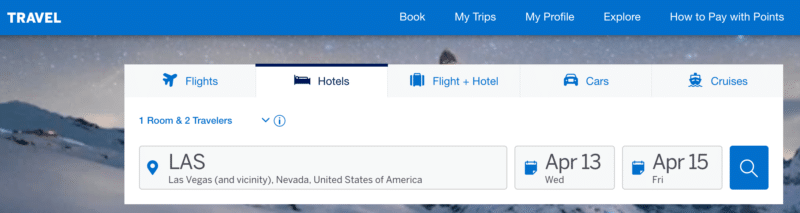A small screenshot of a web page showcases a predominantly royal blue header. In the header, prominently on the left side in bold, white, capital letters, is the word "TRAVEL". Towards the middle to the right, white text aligns horizontally, reading: "Book My Trips," "My Profile," "Explore," and "How to Pay with Points."

Below the header, the page's background transitions to show an image depicting serene snowfall, with a starry or snowy sky above and snow-covered ground below. Slightly to the right of the center is a white rectangular box. In the box, the text and elements appear neatly organized.

At the top of the white box, there is a row featuring five tabs with icons and text: the first tab labeled "Flights" with an airplane icon, the second tab "Hotels" with a bed icon (highlighted in dark blue or black), the third tab "Flight + Hotel" with a suitcase icon, the fourth tab "Cars" with a car icon, and the fifth tab "Cruises" with a ship icon.

Below this row, on the left side of the box, text reads "1 room, 2 travelers" in blue, accompanied by a down arrow and an information icon (a circle with an 'i' in it). Towards the bottom of the white box, another row of tabs begins. From the left, the first tab shows a location pin icon next to "LAS Las Vegas and vicinity, Nevada, United States of America." The middle box indicates the date "April 13th (Wednesday)," and the third box from the left shows "April 15th (Friday)." 

Lastly, a blue search button featuring a magnifying glass icon is positioned to the right end of this row.